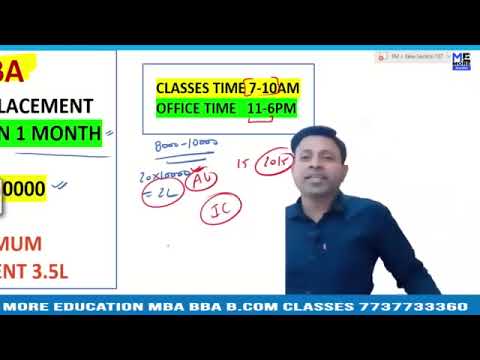This image is a screenshot, likely from an online platform. At the right side, we see a man with a professional demeanor, wearing a blue button-up shirt with a collar. He has short, black hair parted to the left, and his brown-skinned face is partially smiling with his mouth slightly open, revealing his top and bottom teeth. His right arm is angled downwards and out of the frame, overlaid by text.

The background features a bulletin or whiteboard filled with text and diagrams. Prominent at the top left, a yellow section reads "Classes Time 7-10am" in black letters, followed by a green section below that states "Office Time 11-6pm." Both sections include red parentheses emphasizing these times. Below this, there is densely packed text, including handwritten elements, often encircled in red. These details include "equals 2L," "AL," "JC," "15," and a circled "L-O-L-E."

Further to the left, red and yellow sections display "A" in red against yellow, "LACEMENT" in black against white, "N1MONTH" in black against green, "0000" against yellow, "M-U-M" in red against white, and "NT3.5L" in red against white.

Across the bottom of the screen, a blue banner hosts white text that advertises "More Education MBA, BBA, B.com Classes" and provides a phone number, 773-773-3360. At the top and bottom edges of the image, black bars take up additional space, likely acting as borders. In the upper right corner, there is a blue and black decal featuring the letters "M" and "E." This setup suggests that this is a promotional or informational screenshot, possibly for educational courses taught by the man pictured.